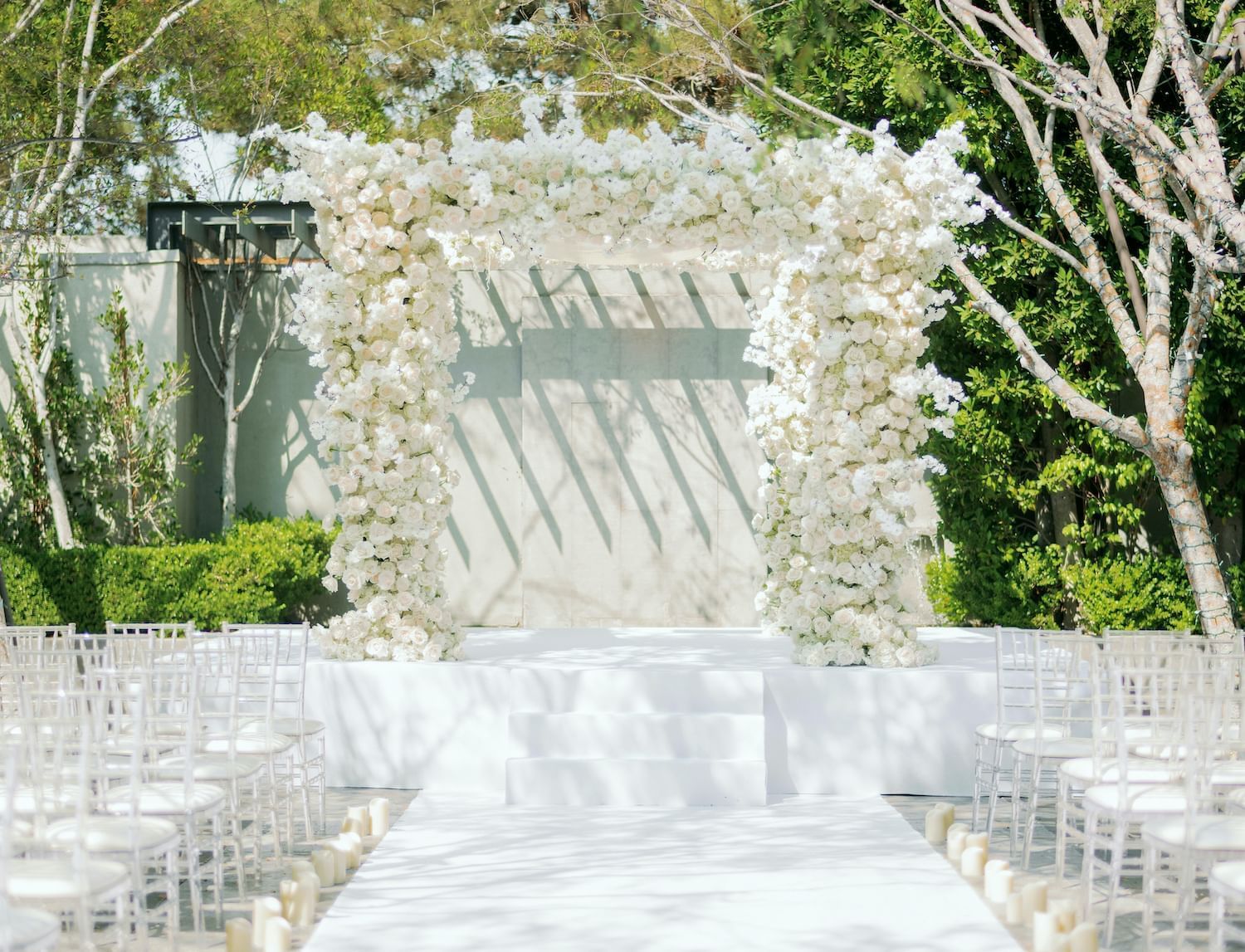This photograph captures an outdoor wedding staging area, likely set in a park or a spacious backyard, bathed in bright daylight. Dominating the scene is a beautifully decorated white altar, featuring an archway intricately adorned with lush white flowers. Leading up to the altar is a pristine staircase composed of three white steps. A white pathway, meticulously bordered by elegant candles, guides the way to the altar. The seating arrangement consists of neatly organized white chairs lining both sides of the path. The venue enjoys a natural backdrop of abundant trees and greenery, adding a serene touch to the festive setup. Additionally, there are distinct pillars and a notable wall in the background contributing to the scenic aesthetic.